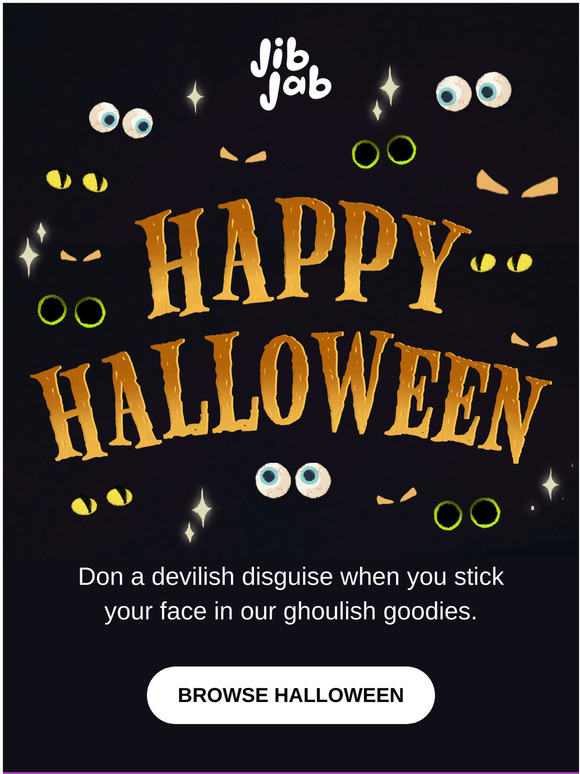The image features a solid black background. At the top of the rectangular frame, the phrase "jib jab" is presented in lowercase letters, with "jab" starting just below the "I" in "jib." The text is styled in a distinct Halloween-themed font.

To the left side of the image, there is a diamond-shaped star, followed by a set of two eyeballs looking towards the right. Below these, there are two yellow eyeballs gazing upwards. Continuing in a counterclockwise direction, the image displays a variety of Halloween-themed elements: multiple diamond shapes, green eyes, orange eyebrows, and more yellow eyeballs. 

Further along, additional diamonds and eyeballs are arranged, with green eyeballs appearing prominently. As you move up the right side of the frame, you encounter a single star, two orange eyeballs, two yellow eyeballs, and another set of two orange eyeballs. 

Near the top center, around the 12 o'clock position, there are two green-outlined eyeballs alongside two orange eyeballs. The text "Happy Halloween" appears in curved orange letters, arching upward slightly before curving down again. Further below, a smaller line of text states, "Don a spooky disguise as you indulge in our ghoulish goodies." This is followed by a white bar at the bottom featuring the text "Browse All Halloween" in black font.

The overall design exudes a festive and eerie Halloween vibe through its use of colors, fonts, and thematic imagery.